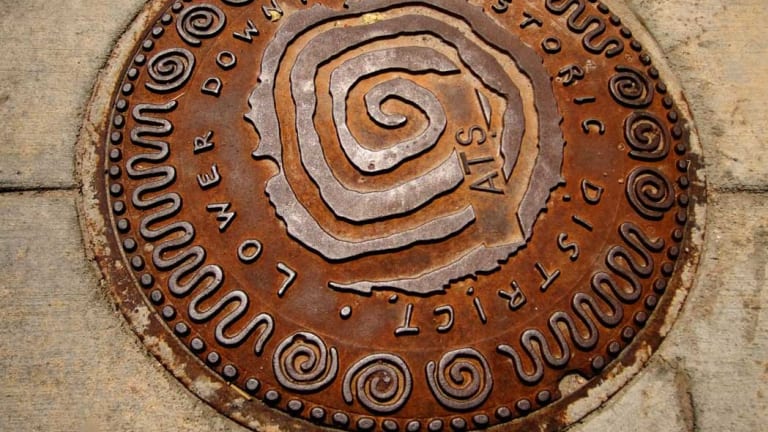The image captures a close-up view of a worn, rust-colored manhole cover, partially embedded in a concrete sidewalk. The cover features a prominent, intricate swirl design at its center, with the capital letters "ATS" prominently displayed within the swirl. Surrounding this central design, there is a semi-circle of text that reads "LOWER DOWNTOWN," likely part of the phrase "HISTORIC DISTRICT," though the word "HISTORIC" is cropped out of the frame. The border of the manhole cover is adorned with a repeated decorative pattern of trios of three swirls connected by curved lines, interspersed with small metal dots that encircle the entire cover. The raised parts of the design and text have a shinier, slightly less rusted appearance, possibly highlighted by a camera flash. The surrounding concrete sidewalk, marked by visible seams, emphasizes the worn and aged character of both the manhole cover and the pavement.